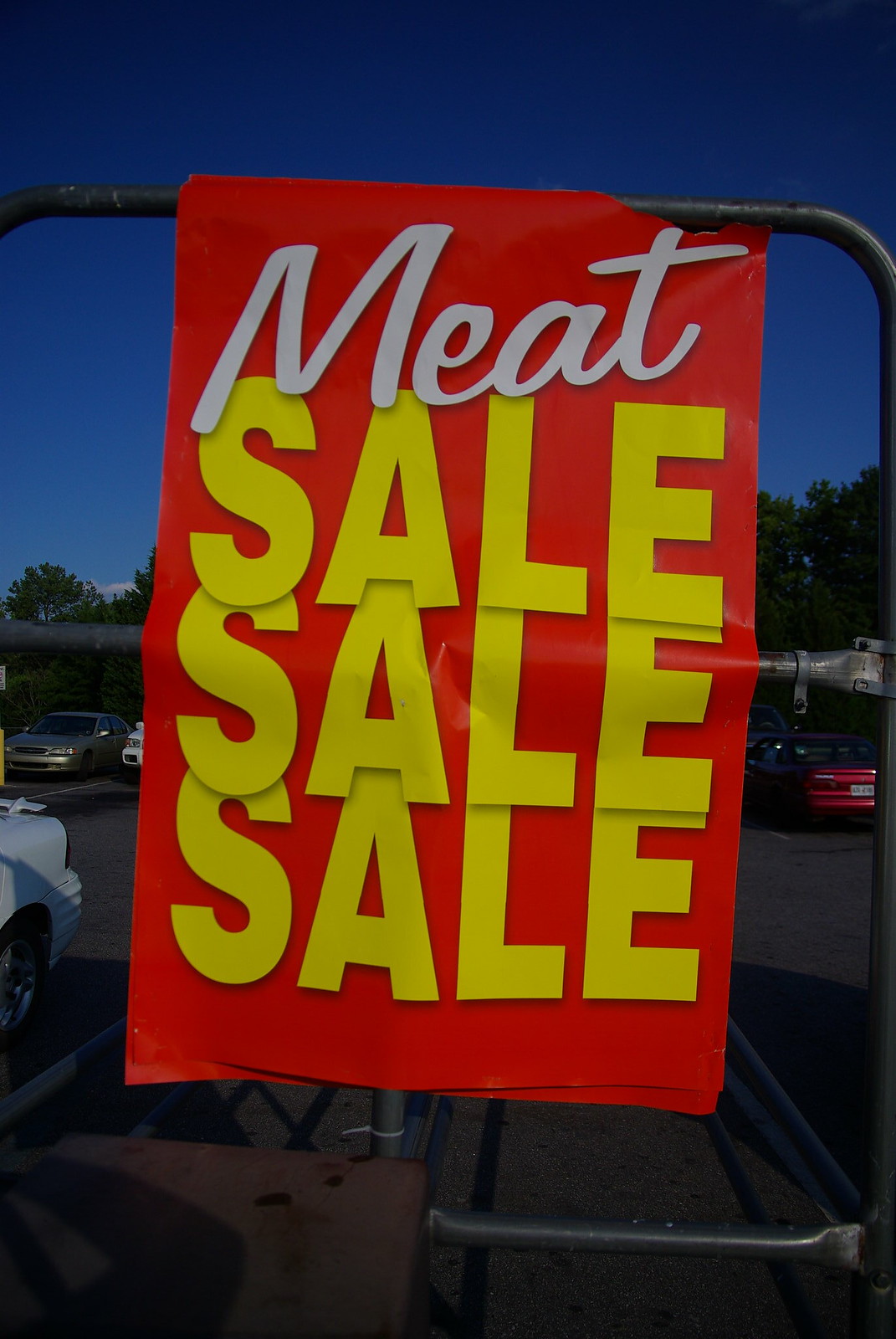A vibrant red banner, displayed prominently on a sturdy metal post, stands out amidst a backdrop of lush green trees. The white text at the top of the banner reads "ME" in bold, attention-grabbing letters. Below this, the word "CELL" appears twice, stacked one below the other. At the bottom of the scene, a paved asphalt road can be seen with several cars parked on it, including one parked to the left of the banner. The overall setting combines natural and industrial elements, emphasizing the banner's message against a dynamic background.